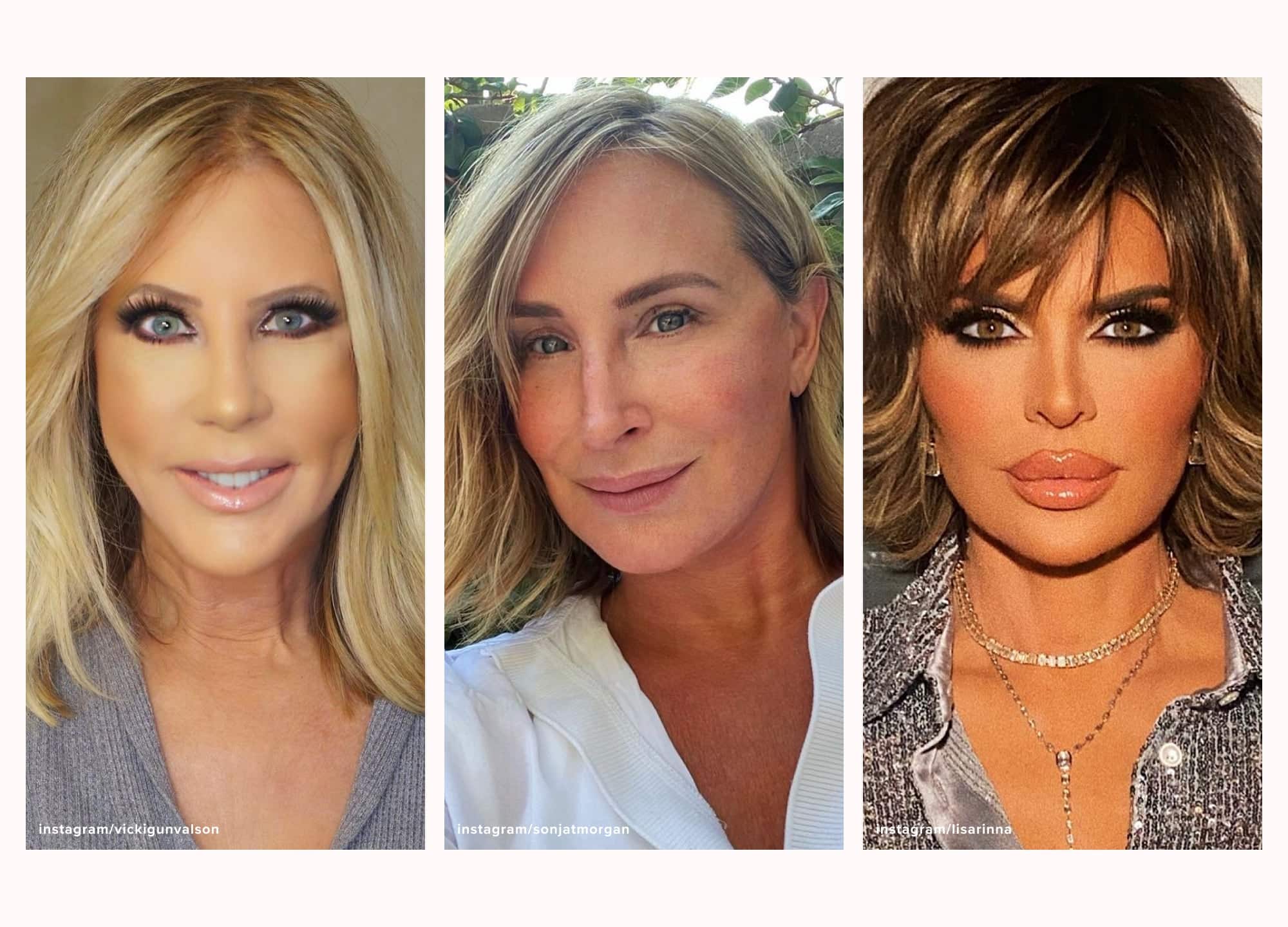The image is a composite of three color photographs placed side by side, each featuring a close-up of a different woman, separated by white lines. The woman on the far left has long blonde hair and blue eyes, wearing a gray sweater and makeup. Her name appears as Vicky Gunvalson underneath her image, next to an Instagram handle. In the middle, there is another woman with long blonde hair, likely Sonya T. Morgan, depicted against a background of green leaves while wearing a white jacket. She appears to be mostly makeup-free. The woman on the right, named Lisa Rina, has short brown and blonde hair, brown eyes, pronounced red lips, makeup with dark eyelashes, and is wearing a gray button-down shirt adorned with necklaces. The photograph captures the head and neck areas of these women, hinting at their potential fame, possibly as actresses.